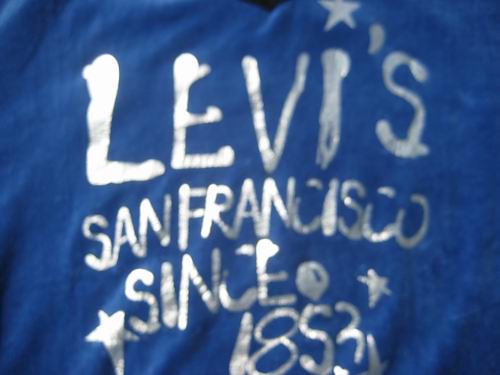Displayed in the image is a large pair of blue jeans hanging upside down. The denim fabric is visibly wrinkled, adding texture to the scene. Prominently written in bold, white letters on the lower legs are the brand name "Levi's." The text utilizes a stylized font, and as a creative touch, a large white star dots the "i". Accompanying the brand name, additional text reads "San Francisco since 1853," with a star positioned beside "since" and another star atop "1853." The lettering appears to have been meticulously applied using a white pen or marker, which stands out vividly against the dark blue of the jeans. This artistic display not only highlights the iconic Levi's brand but also pays homage to its historical roots in San Francisco, dating back to 1853.